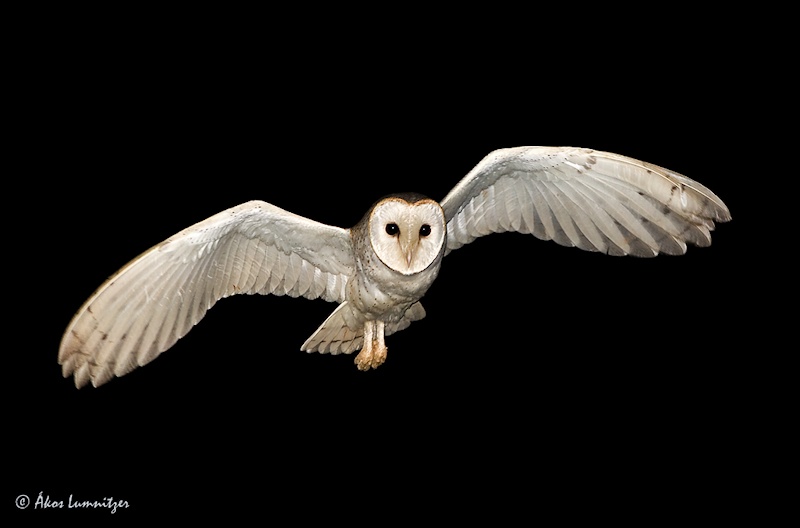This is a striking real-life photograph of a white barn owl in mid-flight, set against a stark, solid black background. The owl is captured with its expansive wings spread symmetrically, creating an impression of majesty and grace. The bird's legs trail behind it, adding to the dynamic sense of movement. Its face is distinctively heart-shaped, characterized by large, expressive black eyes and a beak that forms a V-shape beneath them. While the owl's plumage is predominantly white, subtle shades of beige and hints of gray can be observed, particularly on the tips of its perfectly white wings, contributing to a textured appearance. The photograph is credited to a photographer whose name appears in cursive at the bottom left-hand corner, seemingly starting with "A" and possibly reading "AKOS LUMONITZER," and is marked as copyrighted. The meticulous details and contrast highlight the owl's elegant yet formidable presence.